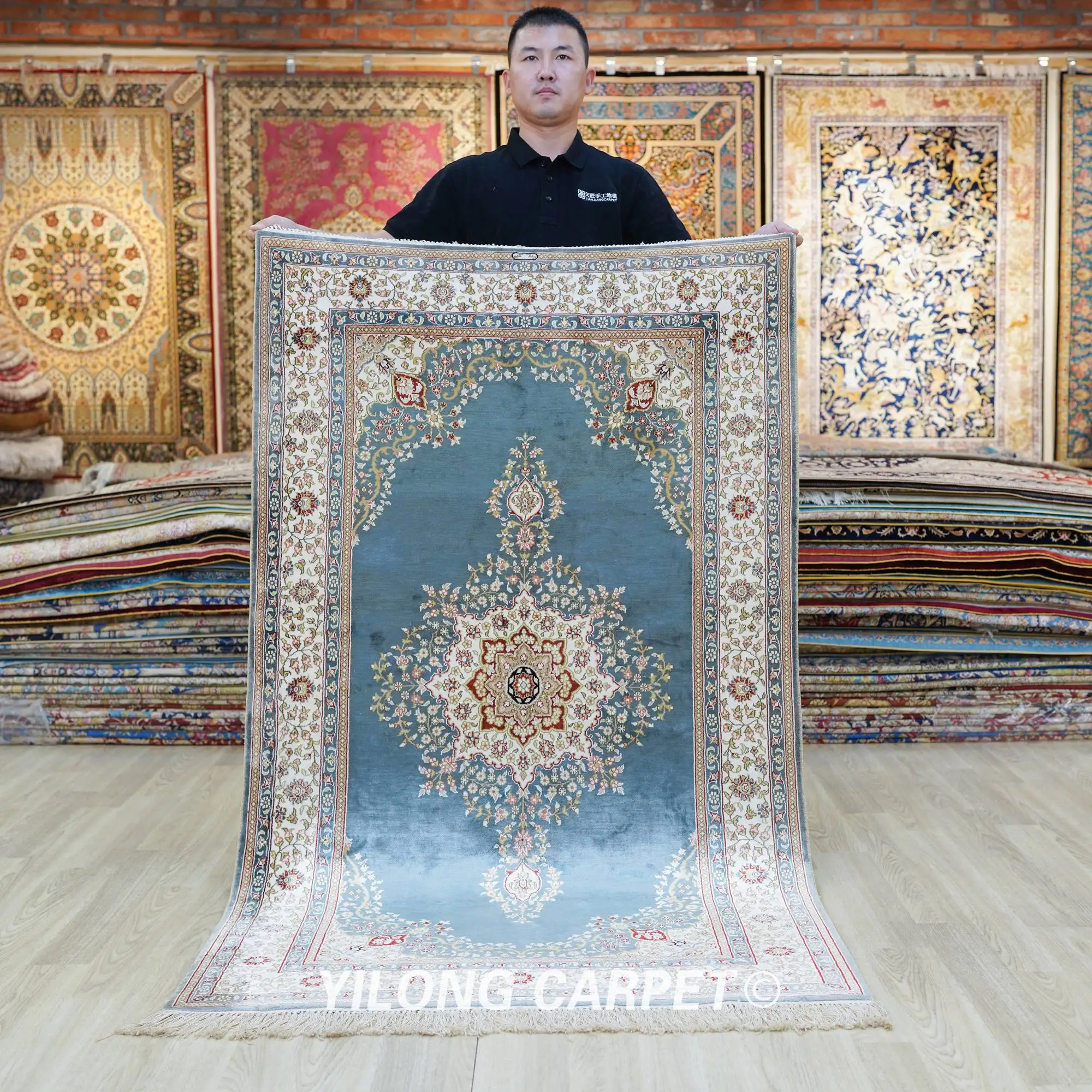In this image, a man of likely Asian descent is standing in a room showcasing a beautifully patterned rectangular rug. He is wearing a black polo shirt with a white logo on the left side of his chest and has short black hair. The rug he holds, using his left and right hands at the upper corners, features an intricate design with blue, red, yellow, gold, tan, and white colors, complete with tassel-like ends. The man is standing on what appears to be a gray hardwood or vinyl floor, and the setting around him includes a variety of rugs both stacked on the ground and hanging vertically against a brick wall. The bottom of the rug he holds displays the text "Yilong Carpet" in white. The detailed rug design exhibits a central pattern surrounded by a rectangular border with additional ornate designs.